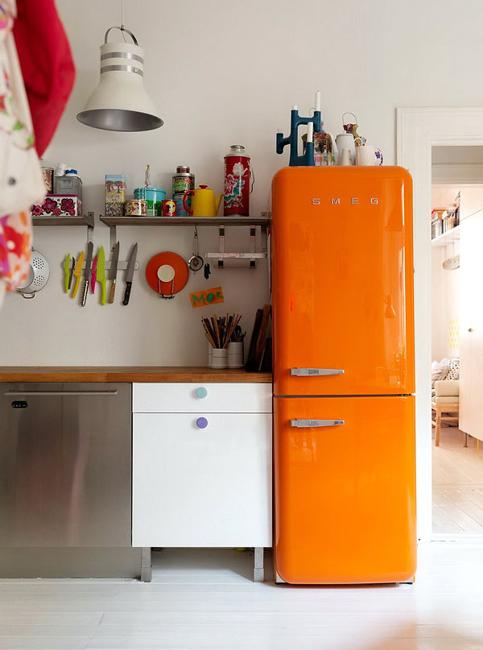This detailed photograph captures a vibrant kitchen scene featuring a striking, bright orange refrigerator with the brand name "S-M-E-G" emblazoned across the top. The refrigerator, which has the refrigeration compartment above and the freezer below, is adorned with silver handles. To the left of the refrigerator stands a white cabinet, comprising a shallow upper drawer and a deeper lower drawer, accompanied by a silver appliance that resembles a dishwasher. Over the white and silver appliance ensemble rests a brown wooden countertop, where bowls with silverware are neatly placed. Adjacent to this arrangement on the wall, multicolored knives—green, yellow, and red—are securely held by a metallic knife rack.

The kitchen floor is pristine white, adding a bright and clean look to the space. Above the countertop is a silver shelving unit filled with various tools, cups, and kitchen items, with additional cutlery and knives hanging beneath it. Bowls and cups are also placed on top of the refrigerator, adding to the clutter and character of the scene. In the top right corner, slightly blurry objects that might be aprons or clothes are hanging, partially obstructing the view. A mixture of modern and cozy elements, like the white and silver lamp above the shelves, underscores the personal touch of this kitchen. 

Peeking through a doorway on the side, there is a glimpse into the next room, revealing what appears to be a couch or chair, along with some shelving, merging the living spaces in a welcoming manner.